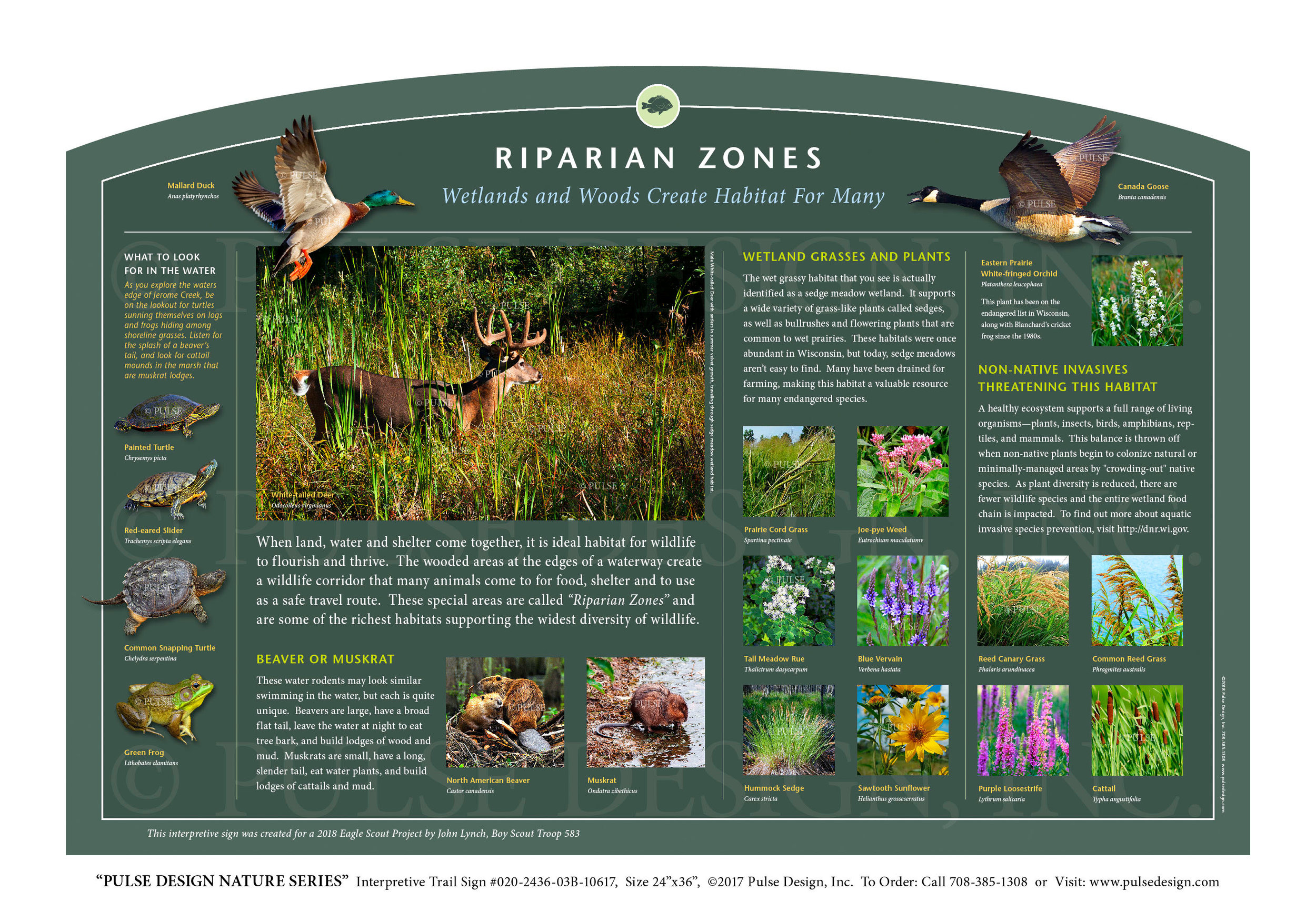The image features a detailed interpretive trail sign from the Pulse Design Nature Series titled "Riparian Zones: Wetlands and Woods Create Habitat for Many." The sign, predominantly dark green with white text, measures 24 inches by 36 inches and describes the critical habitats formed where land, water, and shelter converge.

At the top, the title is in a sans serif font, while the subtitle "Wetlands and Woods Create Habitat for Many" is in a serif style. The upper left corner prominently displays a flying Mallard Duck, characterized by its green head, yellow beak, and orange feet. The upper right corner features a Canada Goose, noted for its black neck, white face, and darker brown wings.

The left side of the sign showcases various wildlife, including:
- Turtles: A snapping turtle with a spiky shell and other species like a painted turtle and a common red-eared slider.
- Amphibians: A green frog with striking black eyes.
- Mammals: A North American beaver and a muskrat.
- Birds: The aforementioned Mallard Duck and other species.

The right side focuses on plant life and non-native invasives:
- Wetland Grasses and Plants: Illustrated with species like hammock sedge, sawtooth flower, prairie cord grass, and tall meadow blue.
- Non-Native Invasives Threatening This Habitat: Featuring plants like reed canary grass and purple loosestrife.

The sign also includes a deer with antlers, standing in a brush of green and brown grasses, symbolizing the diverse wildlife sustained by riparian zones. Additionally, the sign emphasizes the ecological importance of these areas, describing them as some of the richest habitats that support a wide range of wildlife.

At the bottom, the image credits Pulse Design Nature Series, and provides ordering information alongside a 2017 copyright notice for Pulse Design Incorporated.